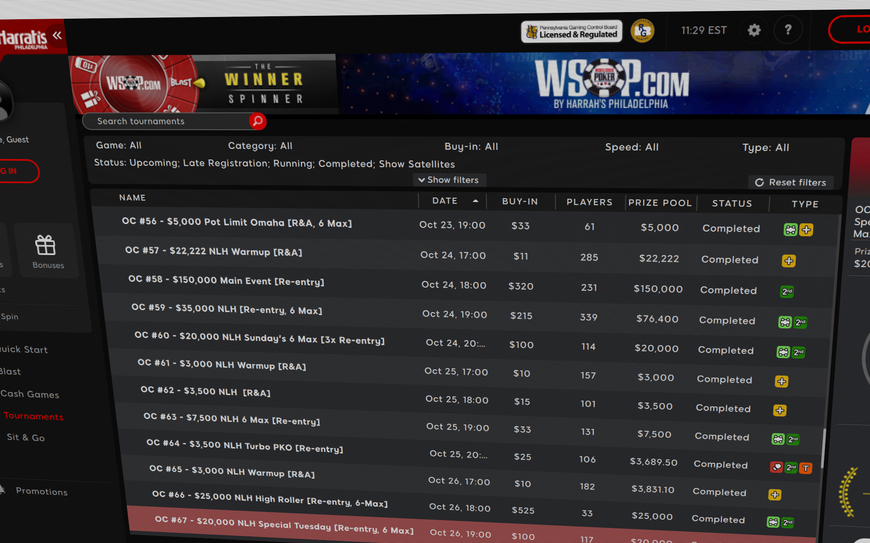The image depicts a webpage for WSOP.com, specifically showcasing the "BLAST - The Winner Spinner" section. At the top of the page, large text reads "WSOP.com" with a logo featuring a black and white poker chip emblazoned with the word "poker." Below this, there is a search bar labeled "Search Tournaments" with a red magnifying glass icon and dropdown options for filtering by "Game," "Category," "Buy-In," and "Status." Status options include "Upcoming," "Late Registration," "Running," "Completed," and "Show Satellites." A "Show Filters" button with a dropdown is also present.

The header also displays "Pennsylvania Gaming Control Board Licensed and Regulated" along with the current time, noted as 11:29 EST.

Underneath, the page lists various tournaments with details such as name, date, buy-in, number of players, and prize pool. For example, the first entry is "OC #56: $5,000 Pot Limit Omaha, 6 Max," which took place on October 23rd at 19:00. The buy-in for this event was $33, and it attracted 61 players, resulting in a prize pool of $5,000. The status is marked as "Completed."

The design includes white text on a gray background, interspersed with various icons and logos, adding splashes of color to the overall layout.